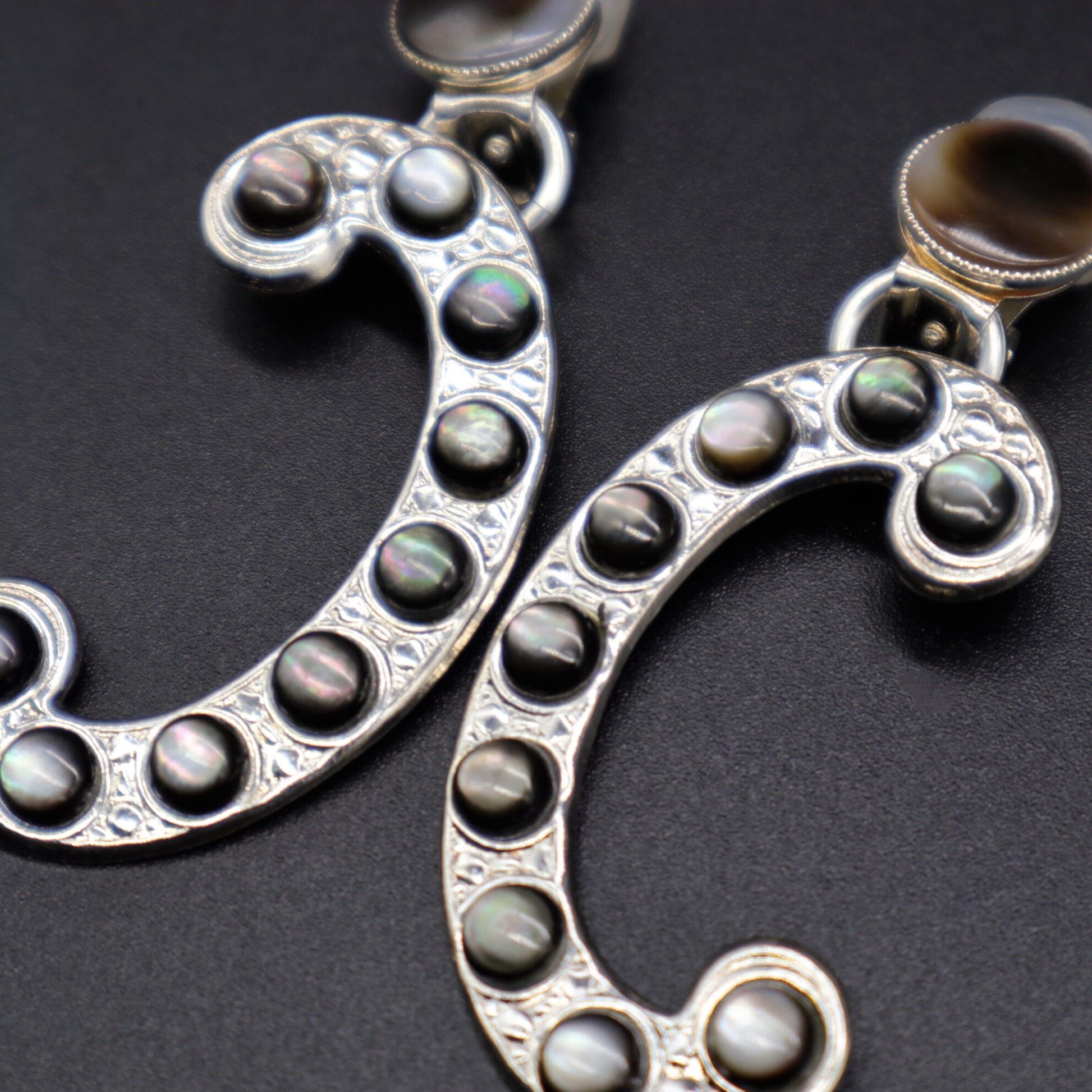This color photograph showcases a pair of intricately designed pierced earrings placed on a textured, dark gray backdrop, potentially resembling a jewelry box or cloth. Each earring features a prominent, smooth circular brown stone at the top, encased in a silver border, with a small silver ring connecting to a larger, dangling pendant. The pendants, crafted from a shiny metallic material in a silver color, are shaped like the letter "C" but oriented differently; one appears as a regular "C" while the other is flipped in the opposite direction. Both "C" shapes are adorned with small dark gray to black stones that have a slight opalescent or iridescent quality, giving the earrings a bejeweled appearance.